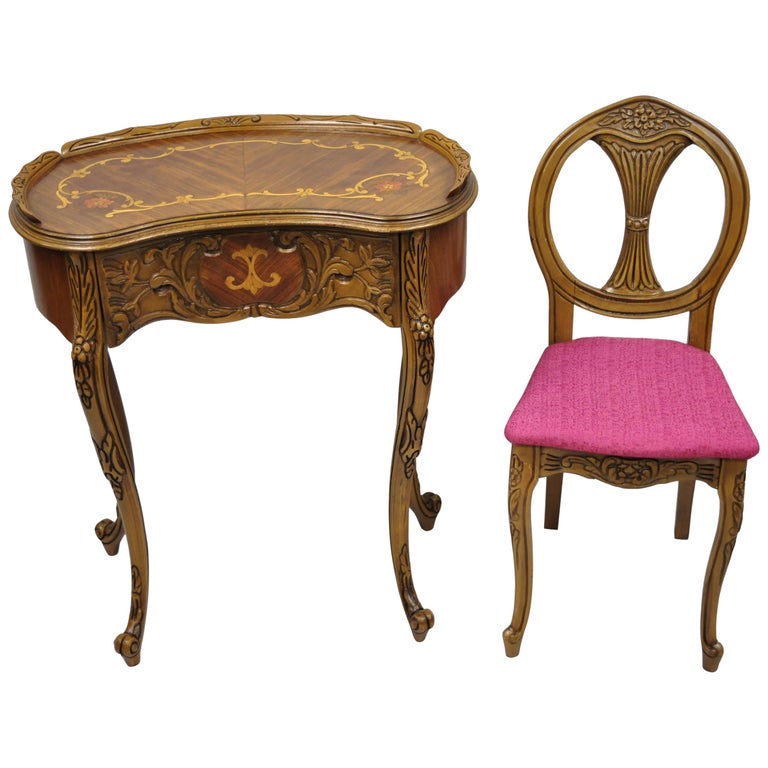This staged photograph showcases two exquisitely detailed antique furniture pieces against a plain white background. On the left, there's an intricately carved oval table with thin, curved legs, each featuring delicate carvings. The table's front has a drop piece with elaborate carvings and an inlaid design. The table's top is adorned with a carved rim encircling an inlaid section with a scalloped, flowery edge. Its rich wood grain is complemented by possibly gold-painted highlights, enhancing its elegance and polished finish.

To the right of the table is a matching chair, sharing the same elaborate design elements and color palette. The chair's front legs curve gracefully, while the back legs are straight. The seat is upholstered in a dark pink fabric. The chair's backrest is oval-shaped with a central wheat straw weave for support and is flanked by two wooden columns. Topping the backrest is an intricately engraved flower motif. This cohesive set, with its harmonious blend of carved details and rich wood tones, presents a regal and timeless aesthetic.